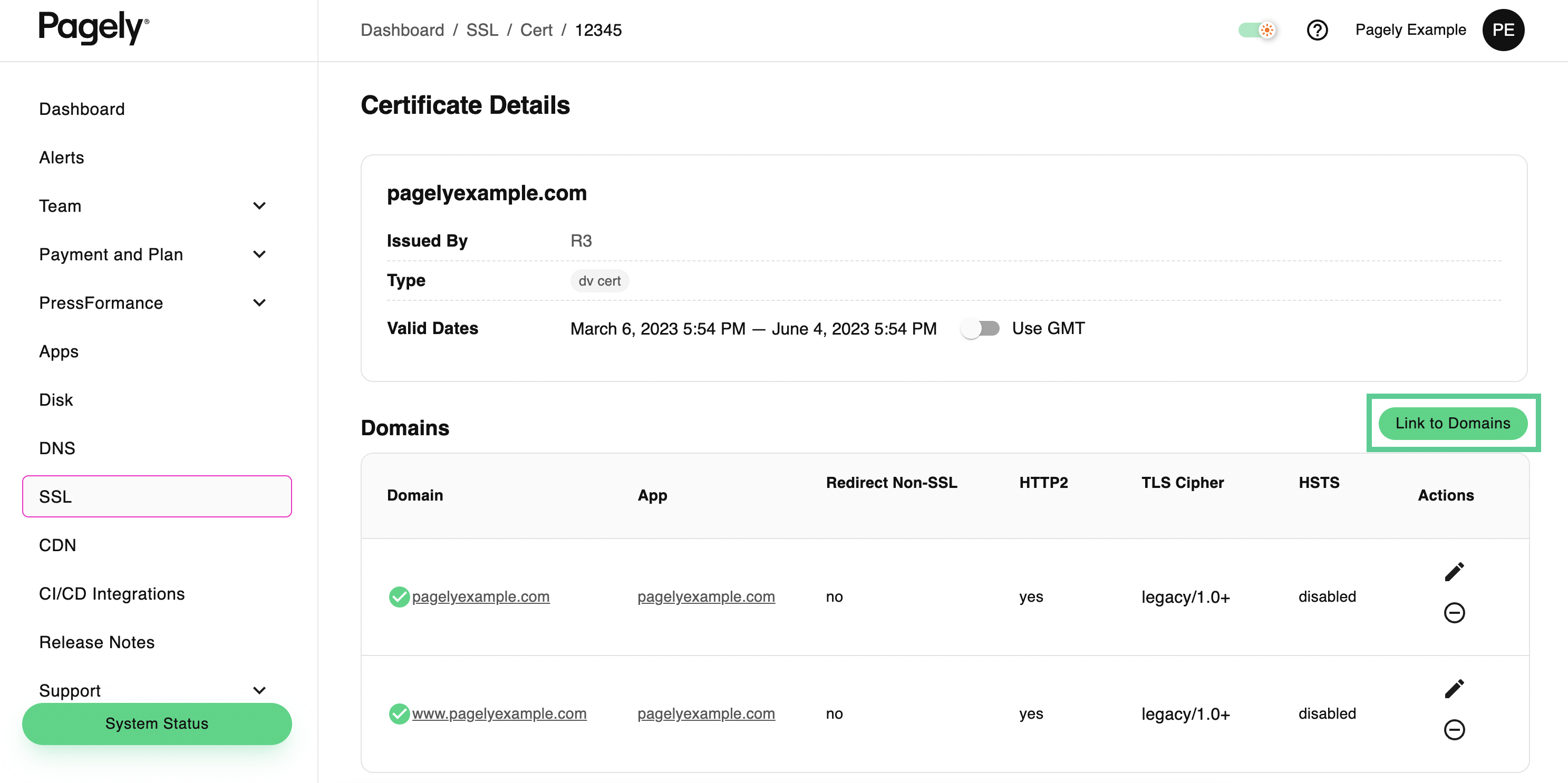Screenshot of Pagely Dashboard: The image showcases a predominantly white dashboard interface from a website called Pagely. In the upper left corner, the Pagely logo is displayed. The left-hand column lists various menu items in black text including: Dashboard, Alerts, Teams, Payment and Plan, Performance, Apps, Disk, DNS, SSL, CDN, CI/CD Integrations, Release Notes, and Support. A prominent green button labeled "System Status" is situated below the menu items.

The main content area of the dashboard is focused on the "SSL" section. Within this section, detailed information about SSL certificates is visible, including certificate details for "pagelyexample.com," issued by R3, with the certificate type specified as DV (Domain Validation) Cert. The certificate is valid from March 6, 2023, to June 4, 2023. Additional subsections under SSL display details about domains, apps, redirects, and non-SSL configurations, filled with technical specifics.